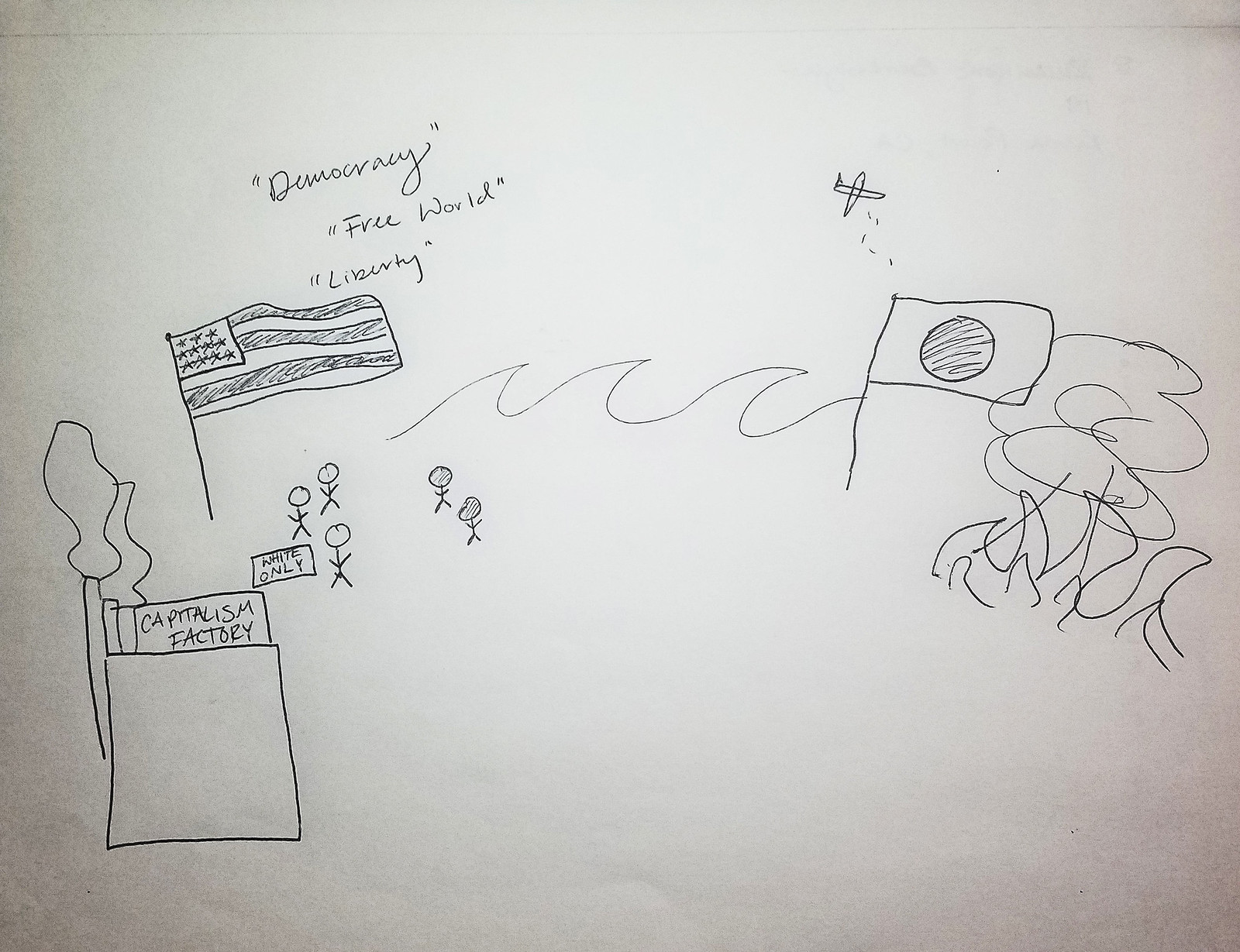The image displays a detailed, hand-drawn scene on white sketch paper using a fine-tip black pen. On the left side of the drawing, there is an industrial building with smokestacks emitting smoke, labeled "Capitalism Factory" across the top. To the right of the factory, three stick figures with blank, white circle heads stand apart from two other stick figures with filled-in, darker heads. A sign between the groups reads "White Only," indicating segregation.

Above them, an American flag is depicted, with the words "Democracy," "Free World," and "Liberty" written in parentheses beneath each term. Below this, ocean waves signify a body of water separating the scenes.

Across the ocean, another flag appears—a rectangle with a filled-in circle at its center. Above this flag, a plane drops items from the sky, which could be interpreted as bombs or supplies. The scene concludes with illustrations of fire and clouds, suggesting explosions or turmoil beyond the horizon.